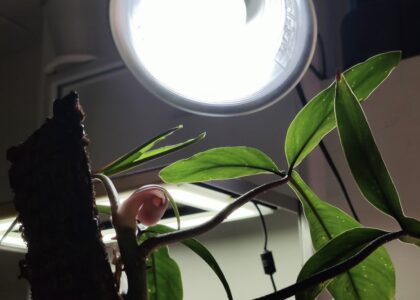This image features a dramatic contrast between light and dark elements. The background is mostly shadowy, with a subtle lighter gradient emerging from the lower right-hand corner. Dominating the left side and center is a vintage desk lamp, showcasing both its incandescent bulb and the reflective dome that houses it. The lamp's power cord trails off towards the lighter gradient, adding a dynamic line to the composition. In the far background, there seem to be additional light sources, possibly featuring a control switch, though it's indistinct and shrouded in darkness.

Foreground elements capture most of the viewer's attention. A climbing vine plant, which might be a syngonium or a philodendron, is prominent. The plant appears to be using a support pole, characteristic of its climbing nature. The leaves form a distinct 'T' shape from the petiole, which is notably substantial, extending back to the main stem. Near the base of this stem, there is visible new growth; it's encased in a thin membrane, tinged red, suggesting its nascent stage. The rest of the image is backlit, casting intriguing shadows and making exact details challenging to ascertain, while the main plant remains the focal point, drawing the viewer into its lush, verdant presence.